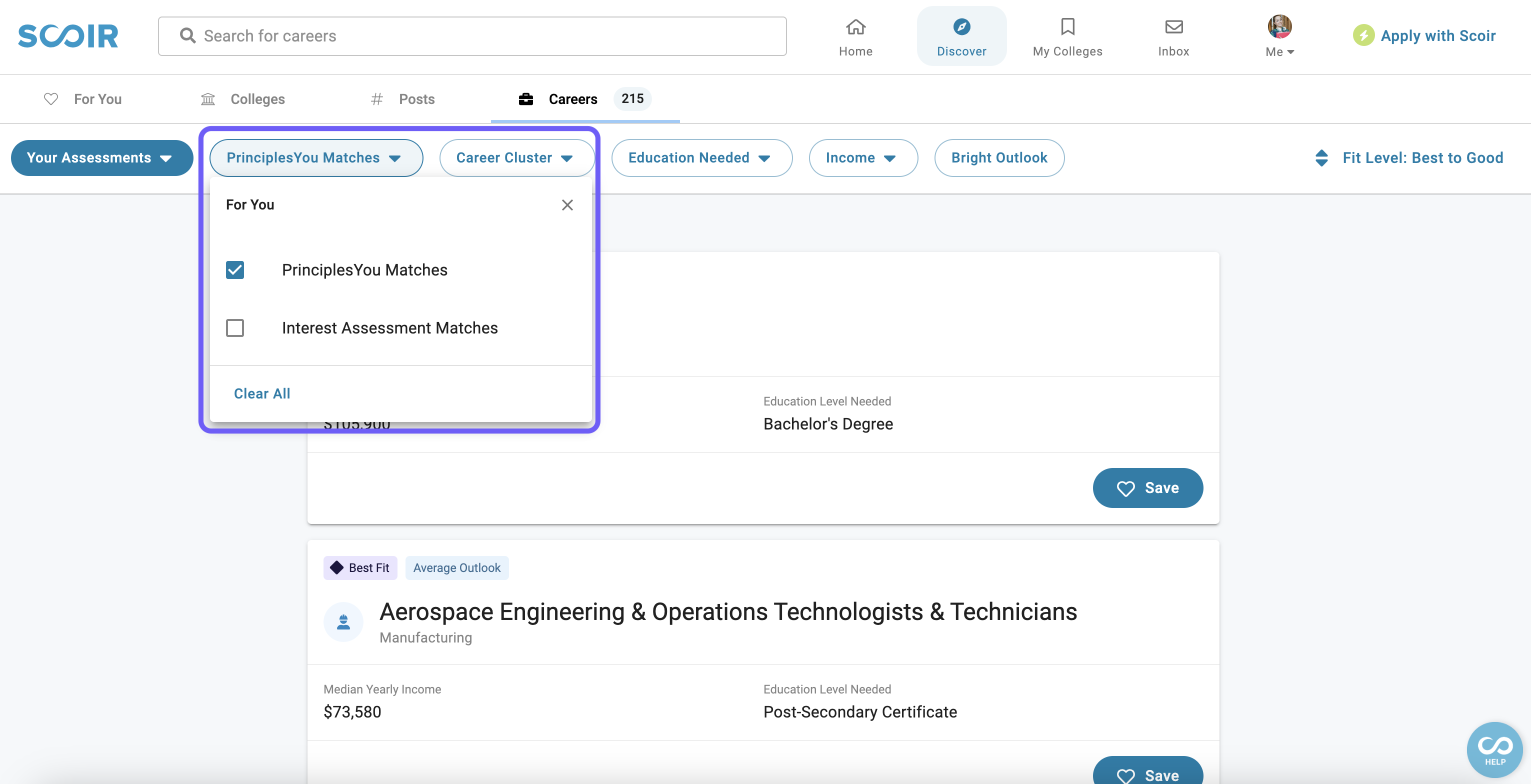The image is a screenshot of a college search website. In the top left corner, the website or company name, "SQUARE," is displayed prominently. Notably, the "C" and "O" in "SQUARE" are stylized as an infinity symbol, resembling a sideways numeral eight, in blue color. At the top of the page, there are navigational elements including a search bar and buttons for "Home," "Discover," "My Colleges," "Inbox," and others.

The main section of the page is focused on a search for college matches. Two primary buttons, "Principles You Matches" and "Career Cluster," are highlighted in purple, indicating their importance. Below these buttons, search results are displayed based on the user's specified interest in a bachelor's degree.

A highlighted section titled "Best Fit" features a specific career match for "Aerospace Engineering and Operations Technologists and Technicians." Accompanying this career title is information on the median yearly income, which is $73,580, and the education level required, identified as a post-secondary certificate.

Overall, the page functions as an advanced search engine, designed to help users fine-tune their college search based on their desired majors and to provide insights into potential earnings and educational requirements after graduation.